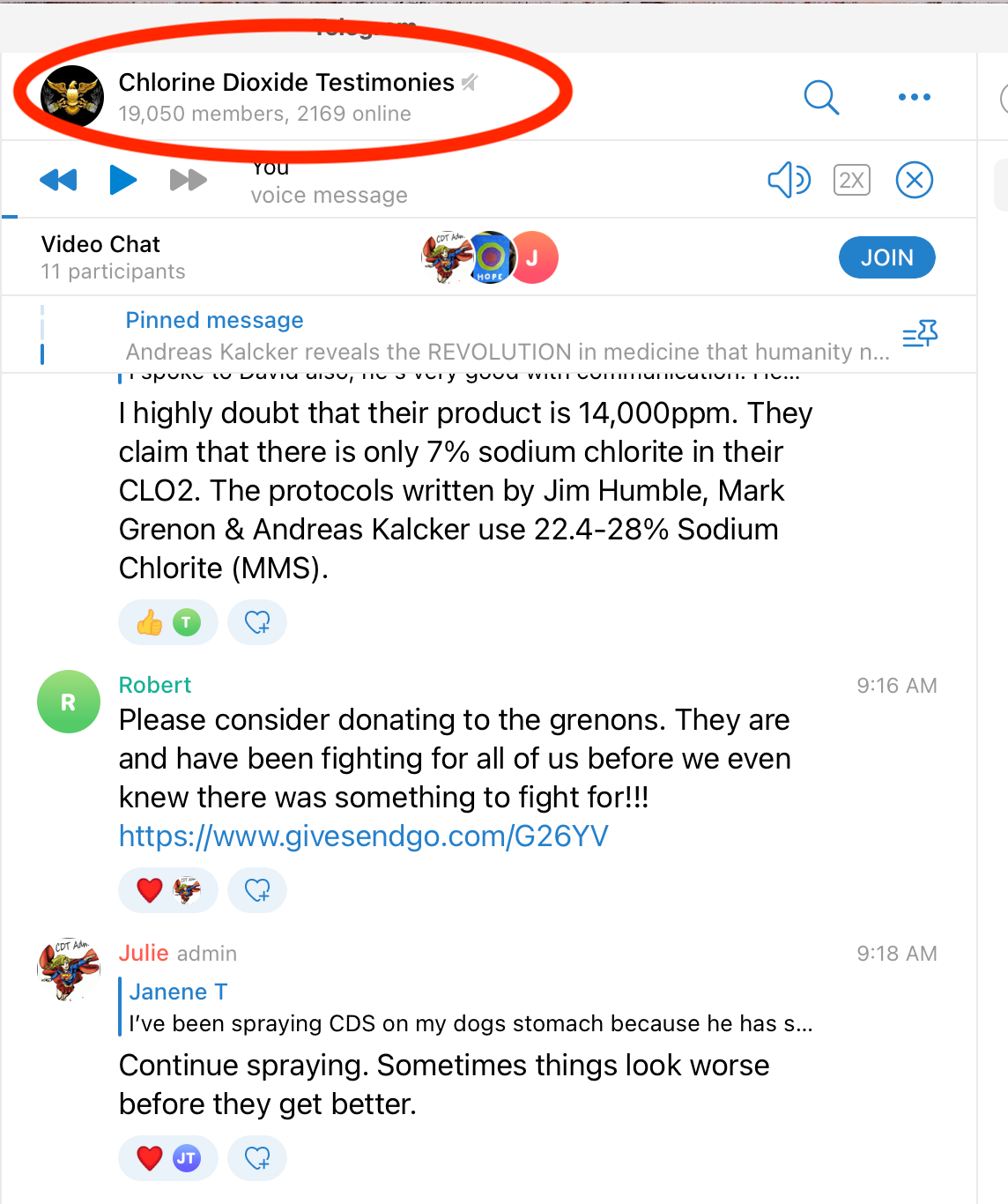This image captures a screenshot of a social media group named "Chlorine Dioxide Testimonies," which appears to be a dedicated forum discussing various aspects of Chlorine Dioxide usage. The group's profile picture is indistinct, displaying an unclear image rather than a person's face. The group boasts a substantial following with 19,050 members, 2,169 of whom are currently online.

At the top of the group page, prominent pinned messages and discussions are visible. One notable pinned post is titled "Andreas Kalker Reveals the Revolution, the Medicine, the Humanity, and ..." with the remaining part of the title truncated, hinting at an in-depth discussion led by Andreas Kalker.

Beneath the pinned post, the screenshot displays snippets of various member posts. One post criticizes the product's claim of 14,000 ppm concentration and questions the accuracy of the sodium chloride content stated as 7% in their Chlorine Dioxide solution. The protocol referenced in the post is associated with Jim Humble, Mark Rennan, and Andreas Kalker, who recommend using a 22.4 to 28% sodium chloride solution, also known as MMS. This post has garnered at least one like.

Further down, a post made by a member named Robert at 9:16 a.m. is visible. Another post follows from Julie, the admin, at 9:18 a.m., where she responds to a query from Janine T. Julie advises, "Continue spraying. Sometimes things look worse before they get better," and her comment has received a heart emoji in response.